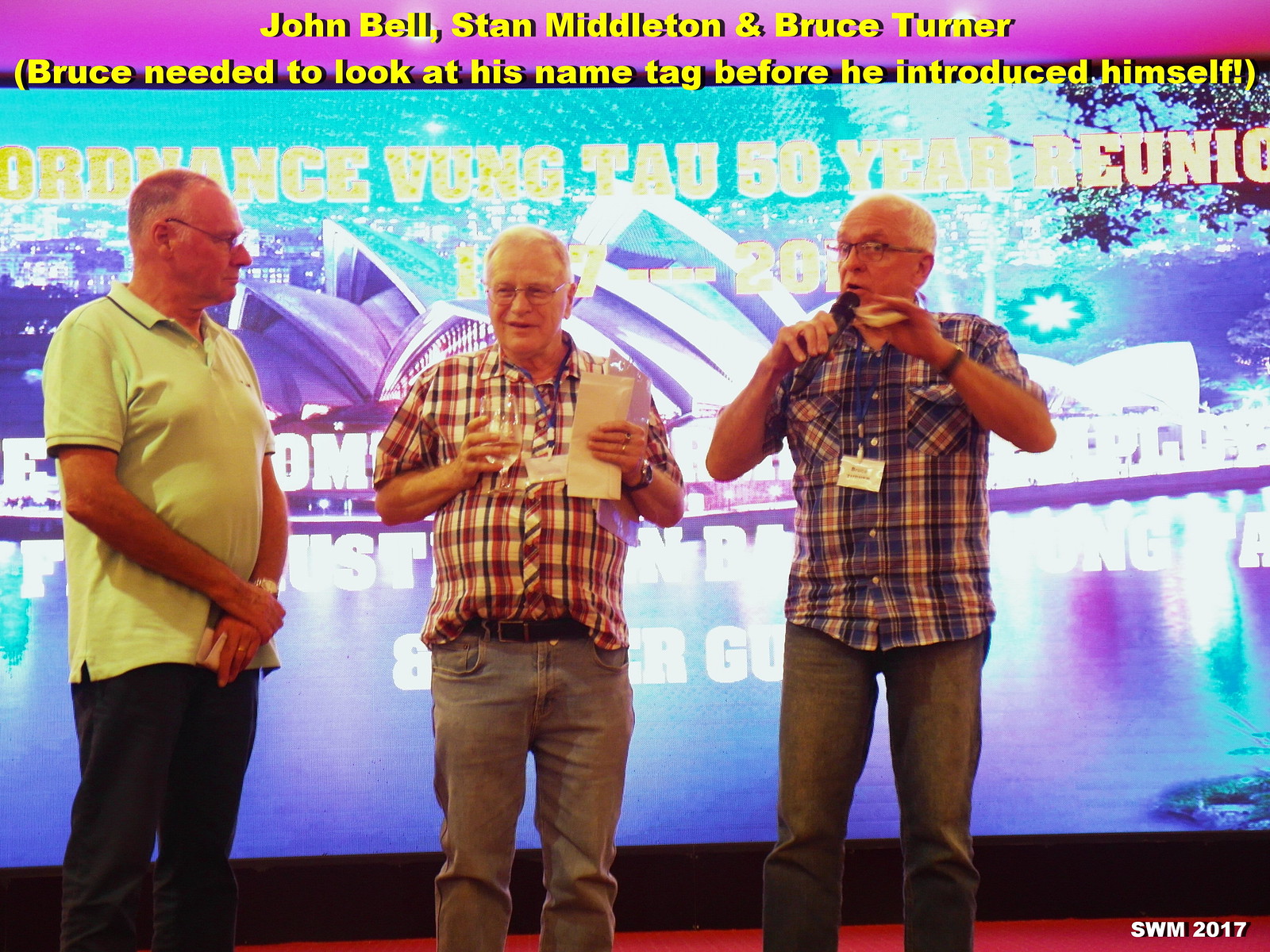This image captures a scene from an indoor event, likely a presentation at a conference or a reunion, featuring three elderly men who appear to be in their early 70s. Positioned directly in the center of the image, the men stand on a red-floored stage in front of a digital screen displaying various colors including red, black, blue, yellow, green, purple, light blue, pink, and gray. The screen's text at the top identifies them as John Bell, Stan Middleton, and Bruce Turner, with a note that Bruce needed to look at his name tag before introducing himself. The screen also includes partially legible information indicating a 50-year reunion, possibly related to an organization abbreviated as SWM, dated 2017.

The man on the far right holds a microphone and is dressed in a short-sleeve blue, red, and white plaid shirt with blue denim jeans. The middle gentleman, also in his early 70s and wearing glasses, holds a piece of paper and a glass of water. He is dressed in a shirt with a similar red, white, and blue pattern and blue jeans. The man on the far left sports a green short-sleeve, collared shirt paired with black pants. Their attire suggests a casual yet coordinated effort, adding to the event's collegial atmosphere.